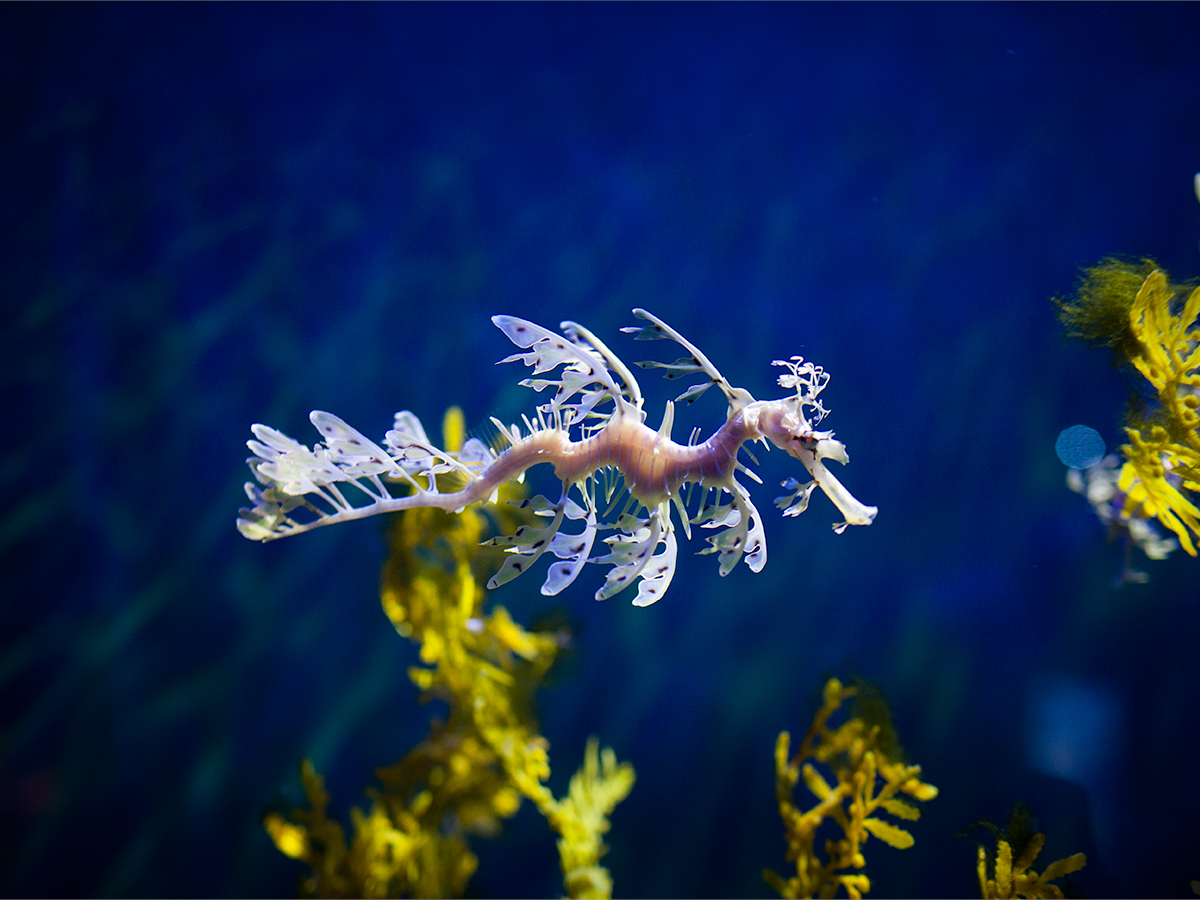This high-resolution underwater photograph captures a mesmerizing sea creature swimming horizontally, facing to the right, in a deep and well-lit, dark blue ocean setting. The background is suffused with an ethereal ambiance created by the interplay of light and rippling water, accentuating the various shades of blue and the blurred, gauzy sea vegetation. Prominent among the flora are four sprigs of almost lime green plants and elements of a coral reef.

In the foreground, the enigmatic sea creature commands attention with its almost otherworldly appearance. Resembling a delicate, fairy-like seahorse, its body radiates a soft, pinkish-white hue. Intricate details abound, as feathery, wing-like appendages—reminiscent of the seed pods from poplar trees—adorn its form, giving the impression of ethereal, fluttering wings. Additionally, the creature features tentacle-like extensions emanating from its face, adding to its fantastical charm. The center of its body showcases a blend of pink and purple tones, interlaced with lines that shimmer with hints of silver or black, contributing to the striking, magical aesthetic of this captivating underwater scene.